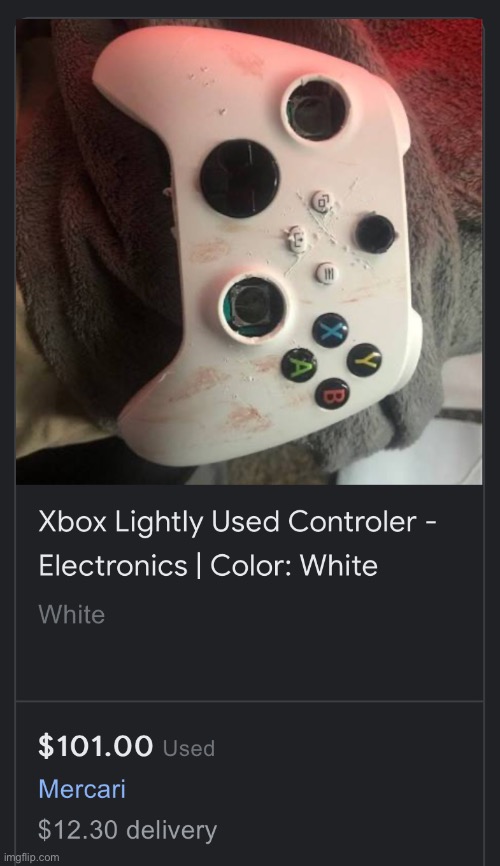A heavily scuffed and scratched white Xbox controller, listed as "lightly used," is featured in a sale on Mercari. The controller has significant damage, including broken analog sticks and overall wear indicative of extensive use. The listing specifies the item is under the "electronics" category. The price is set at $101 with an additional $12.30 for delivery. The Mercari logo is prominently displayed in blue. The entire background of the image is black, with a watermark from imageflip.com at the bottom.